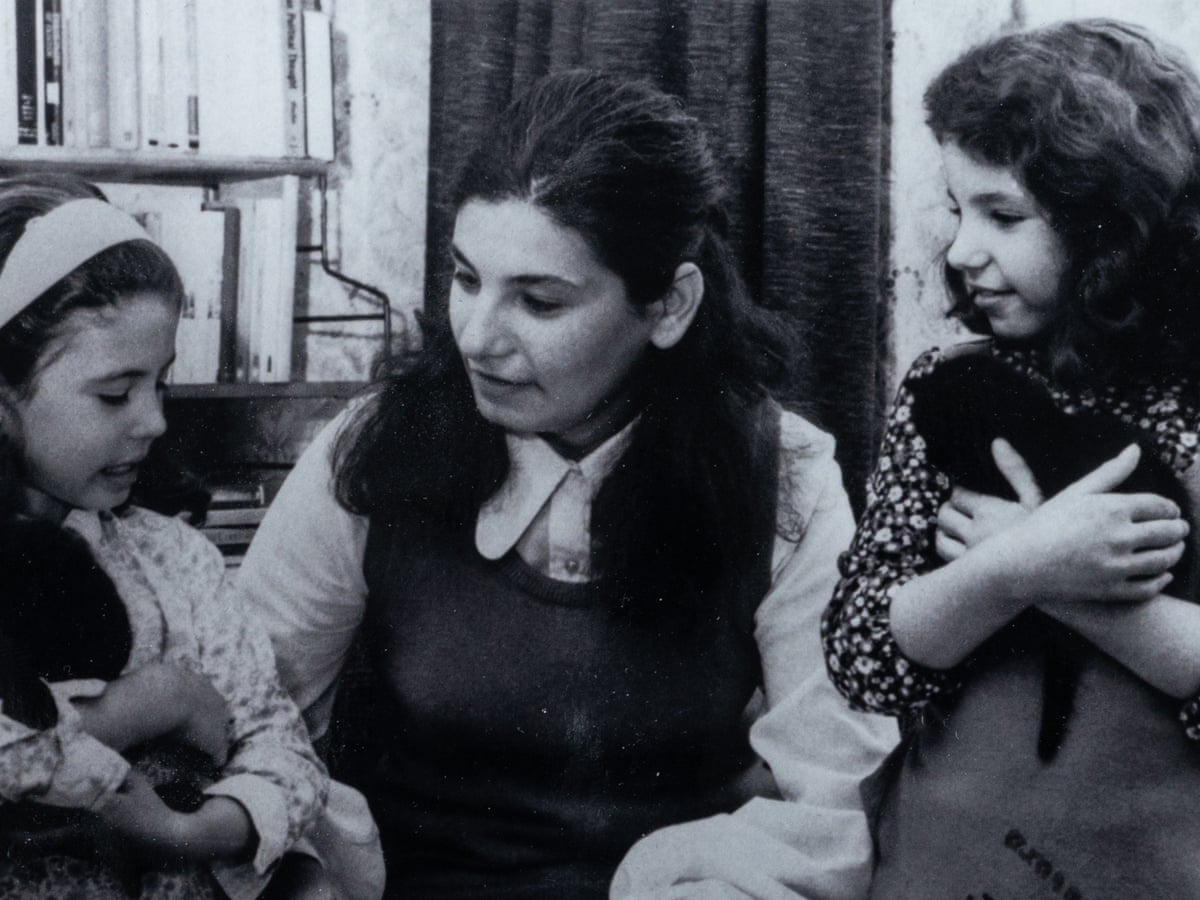This black and white photograph, slightly faded and taken indoors, captures a poignant moment of interaction between a woman and two young girls, both around eight years old. The woman, possibly in her late 30s or 40s, has long dark hair tied back in a half-up, half-down style. She wears a white shirt with a dark sweater vest over it. To her left, a girl with a white headband and dark hair, dressed in a floral print dress with long sleeves, holds a small black kitten in her arms while looking up at the woman. On the woman’s right, another girl with puffy dark hair in a floral top and possibly a pinafore dress observes the interaction, also cradling a black kitten. The setting appears to be an office or a room with a desk, shelves filled with books, and a curtain in the background. The woman and the girls, engrossed in their interaction, subtly reflect an era reminiscent of the 1960s or 70s.